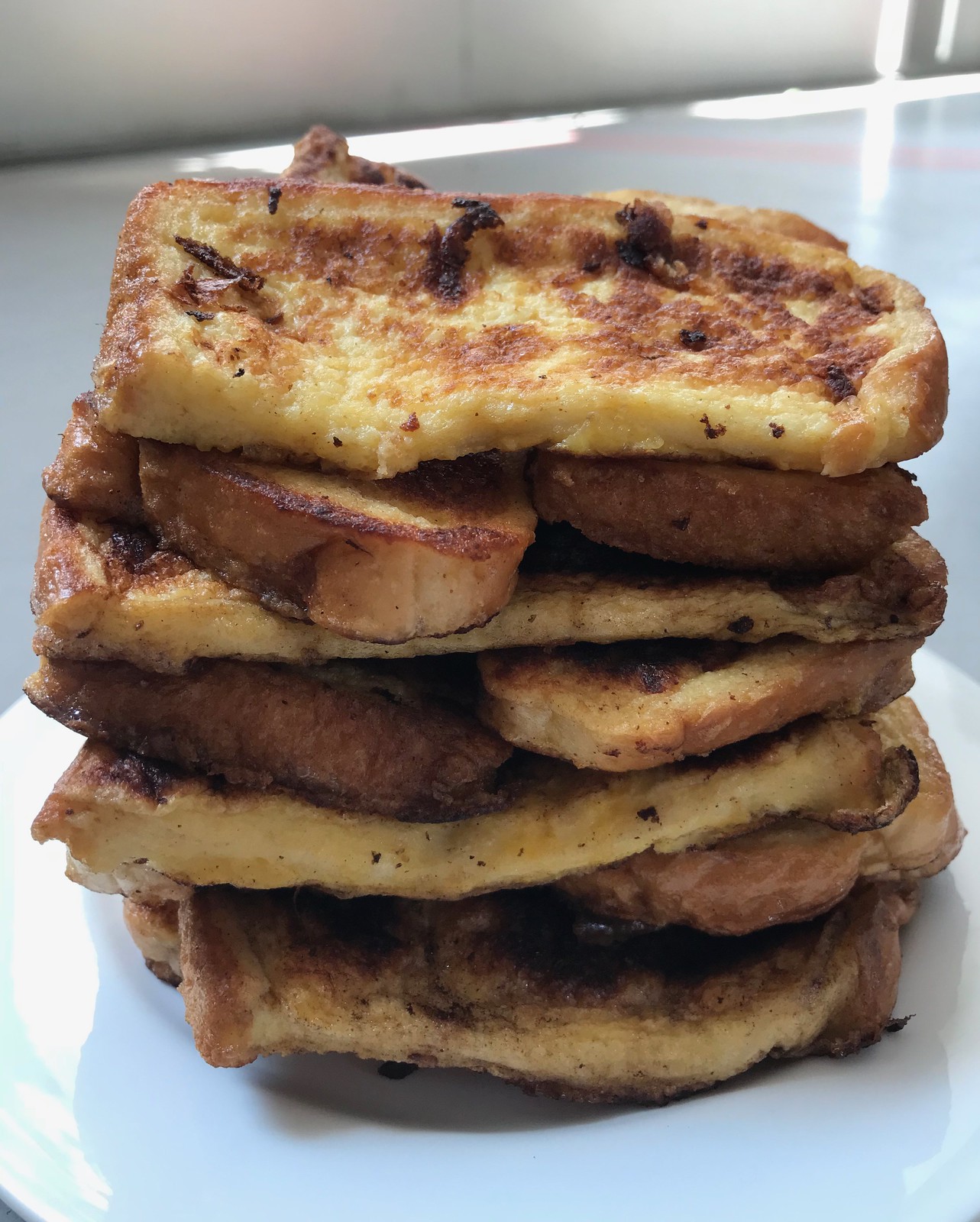In the image, a stack of what appears to be French toast is piled high on a pristine white ceramic plate, which reflects light from a sunny environment. The French toast features a slightly yellow middle with crisp, browned edges, and is dotted with small black flecks throughout. The stack comprises around eight layers, with some pieces exhibiting darker, almost blackened patches. The top piece also has noticeable blacker bits. The background is a blurred off-white surface, possibly a table or the ground, faintly accented by a red line. The scene is brightly lit, suggesting that sunlight is streaming in from behind.